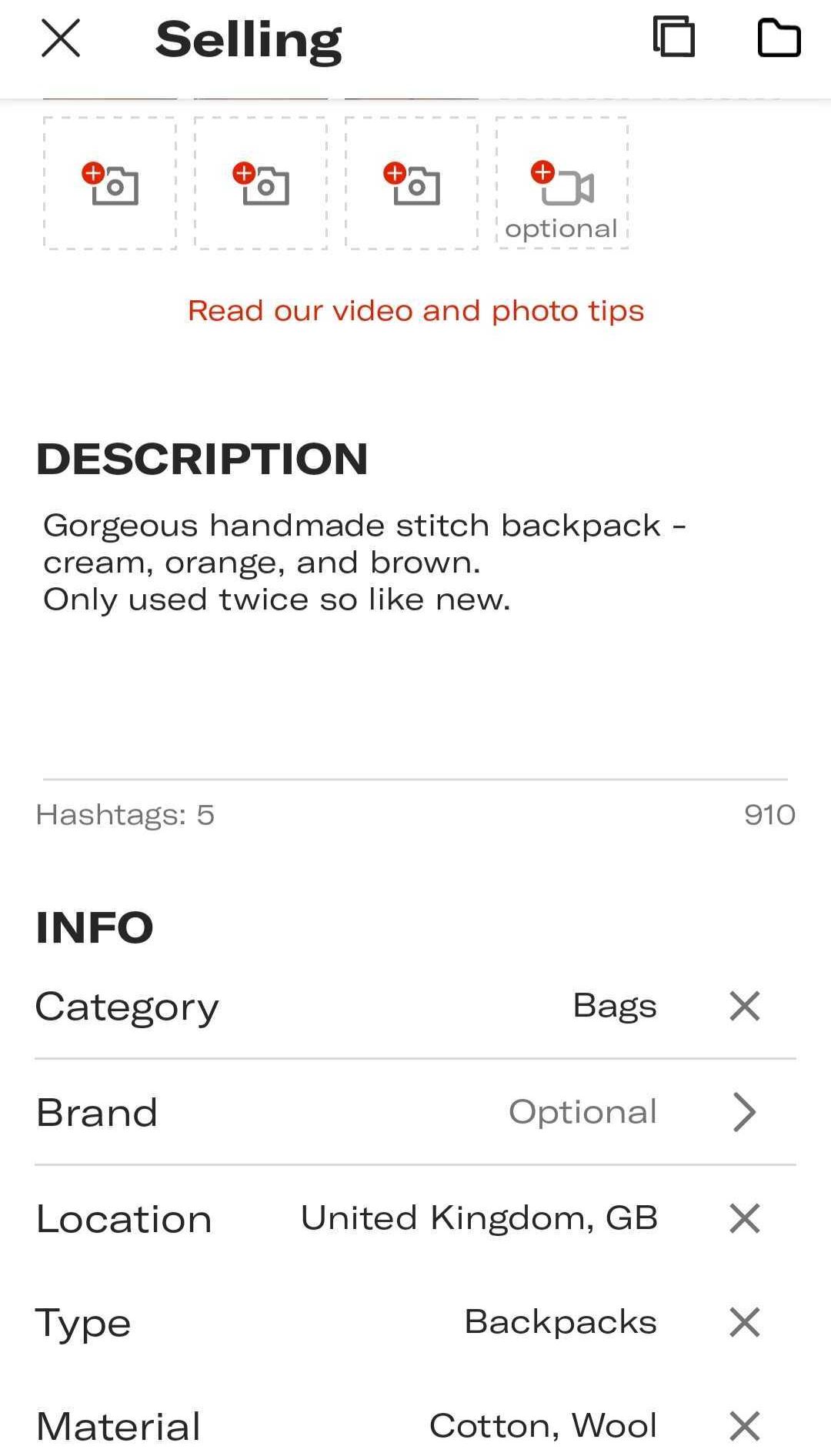The image features a user interface for selling items. At the top, there is a black 'X' icon next to the word "Selling." Additionally, there are icons depicting a couple of sheets of paper and a folder. The upper section has four slots for adding images or videos, each marked with a camera icon – three for photos and one for video, which is labeled "Optional" in grey text. There is also a prompt reading "Read our video and photo tips."

Beneath the section for media, there's a detailed product description: "Gorgeous handmade stitched backpack, cream, orange, and brown. Only used twice, so like new." Five hashtags are also included.

Under the "Info" section, the following details are listed:
- Category: Bags
- Brand: Optional
- Location: United Kingdom, GB
- Type: Backpacks
- Material: Cotton and Wool

Each of these details is accompanied by either an 'X' icon, indicating the option to remove, or a forward arrow, suggesting editability. The design predominantly features a white background with black text, while various functional icons are highlighted in an orange color with notable prominence.